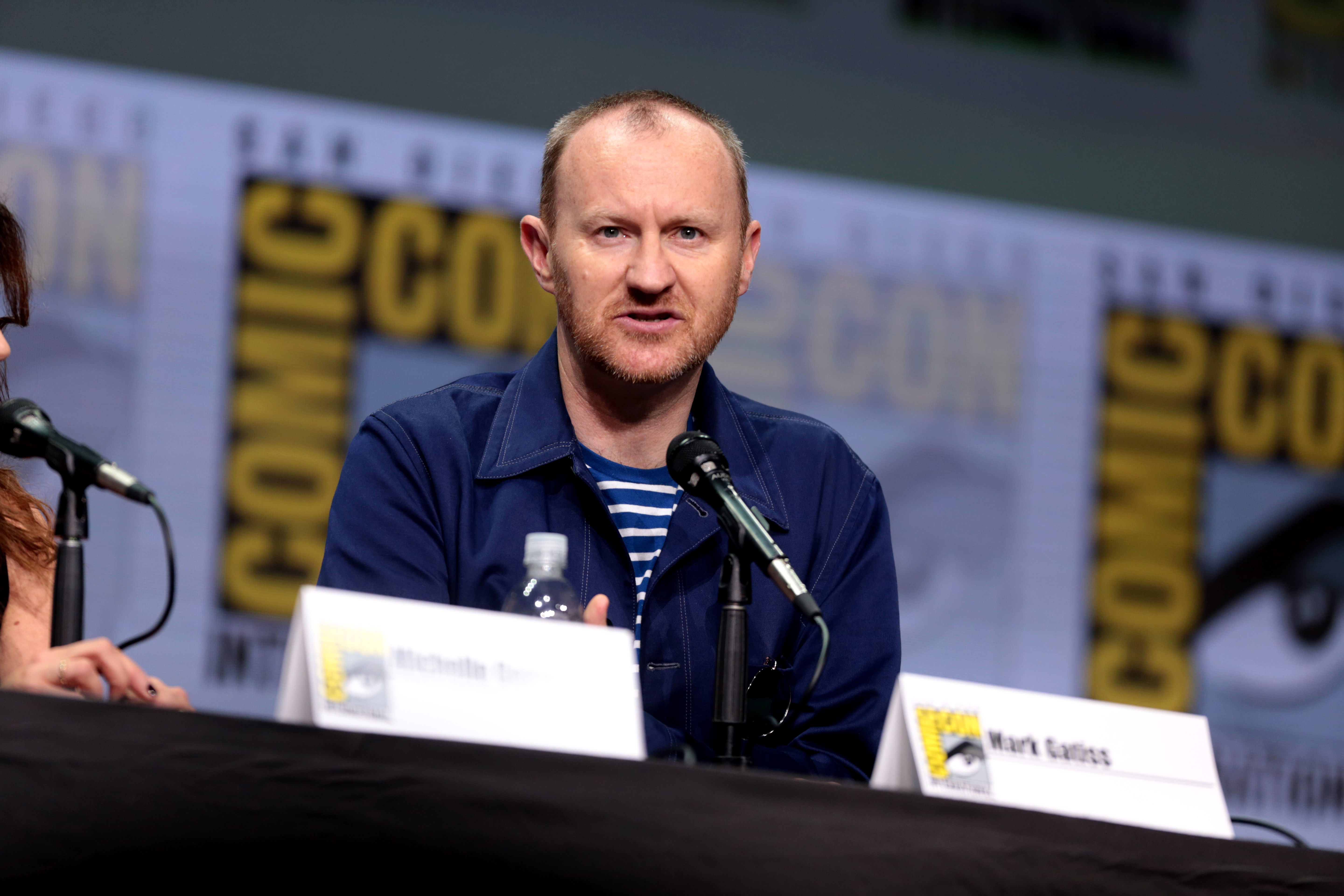In this detailed close-up photograph, we see a bald or nearly bald man with a close-cropped haircut and a receding hairline, wearing a blue jean collared jacket over a blue and white horizontally striped shirt. The man is seated at a table, speaking into a wired microphone that has a black grill top and chrome body with a black cable extending from it. He has a closely shaven beard and mustache with some smattering of facial hair, indicating an in-between stage of grooming. His appearance suggests he is of Caucasian descent, with dark blue or green eyes. His serious and concentrated facial expression indicates that he is in the middle of answering a question, likely during a panel discussion at Comic-Con International, as suggested by the context and partially visible signage in the background. The yellow text that reads "Comic-Con" is rotated 90 degrees counterclockwise, creating an L-shaped angle formation. On the table in front of him, there is a water bottle and a name placard that reads "Mark Kala..." though the last name is not fully discernible. The background also features a partial image of an eye, adding to the Comic-Con ambiance.